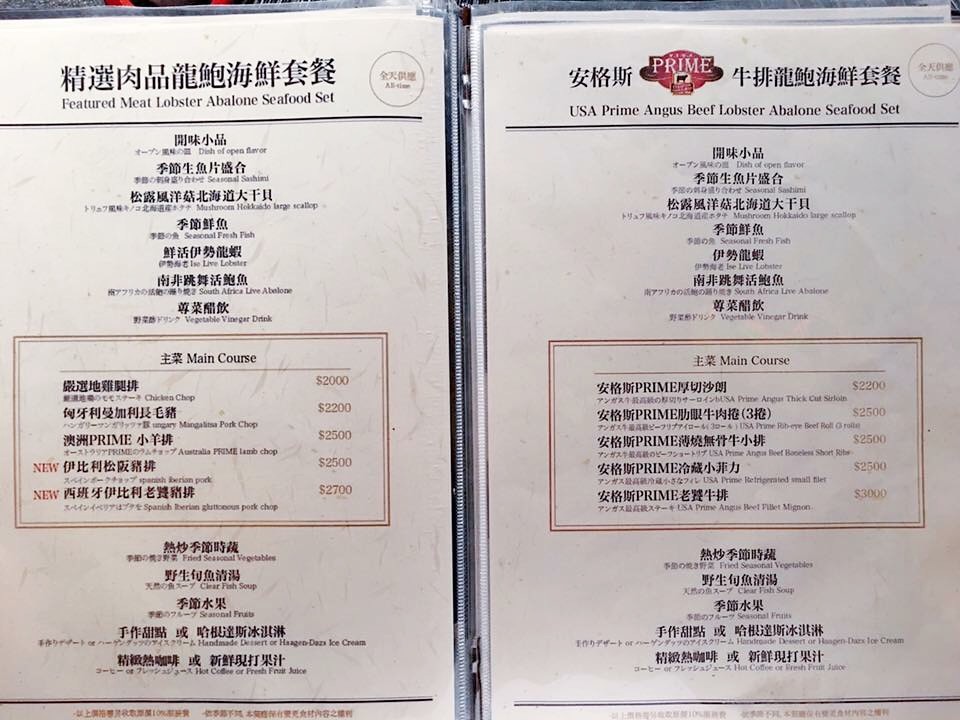The image showcases a high-end, book-style restaurant menu featuring both Chinese and English text. The polished white paper with crisp black text lends an air of sophistication. The left page is entitled "Featured Meat Lobster Avalon Seafood Set," while the right page boasts "USA Prime Angus Beef Lobster Avalon Seafood Set," indicating luxurious seafood offerings. The term "Prime" is prominently displayed, suggesting the use of premium quality meat. The dishes are listed twice on each page—first in Chinese characters and then in English translation, indicating a bilingual menu. The format seems to indicate multi-course tasting menus, possibly with selectable main courses and additional dishes following the main. However, due to the small English print and my inability to read Chinese, the precise details remain partially obscured. Prices for these gourmet meals reach into the thousands of dollars, highlighting the opulence and exclusivity of the dining experience.